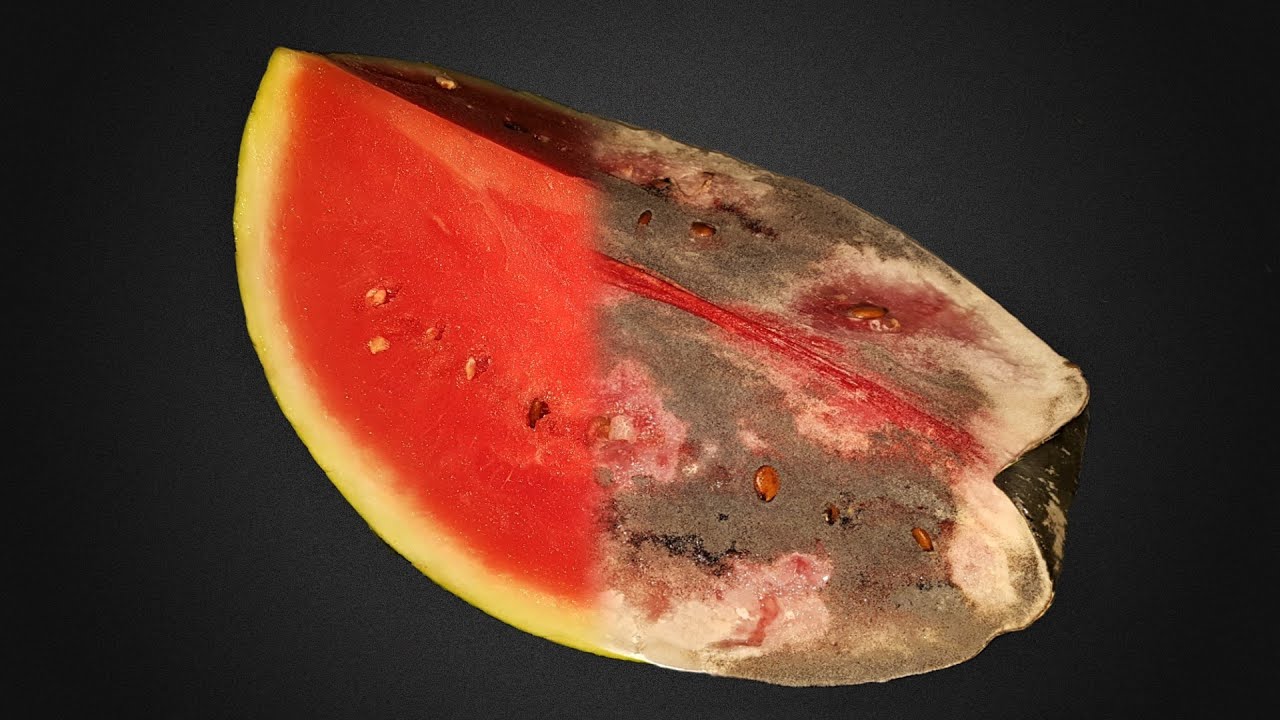The image features a quarter of a watermelon slice laid on its back side, against a solid dark green background. The left half of the slice showcases the fresh, vibrant red flesh of the watermelon, dotted with visible seeds and bordered by its typical bright green rind. In stark contrast, the right half of the slice is covered in decay. The rind has turned dark, almost black, with patches of gray and a painterly-like mold that creates abstract, flower-like patterns. The flesh on the decayed side has lost its vibrant color, displaying unappetizing white and brown spots, and the seeds appear rotten. This juxtaposition between the fresh and rotting sides of the watermelon creates a striking visual dichotomy.